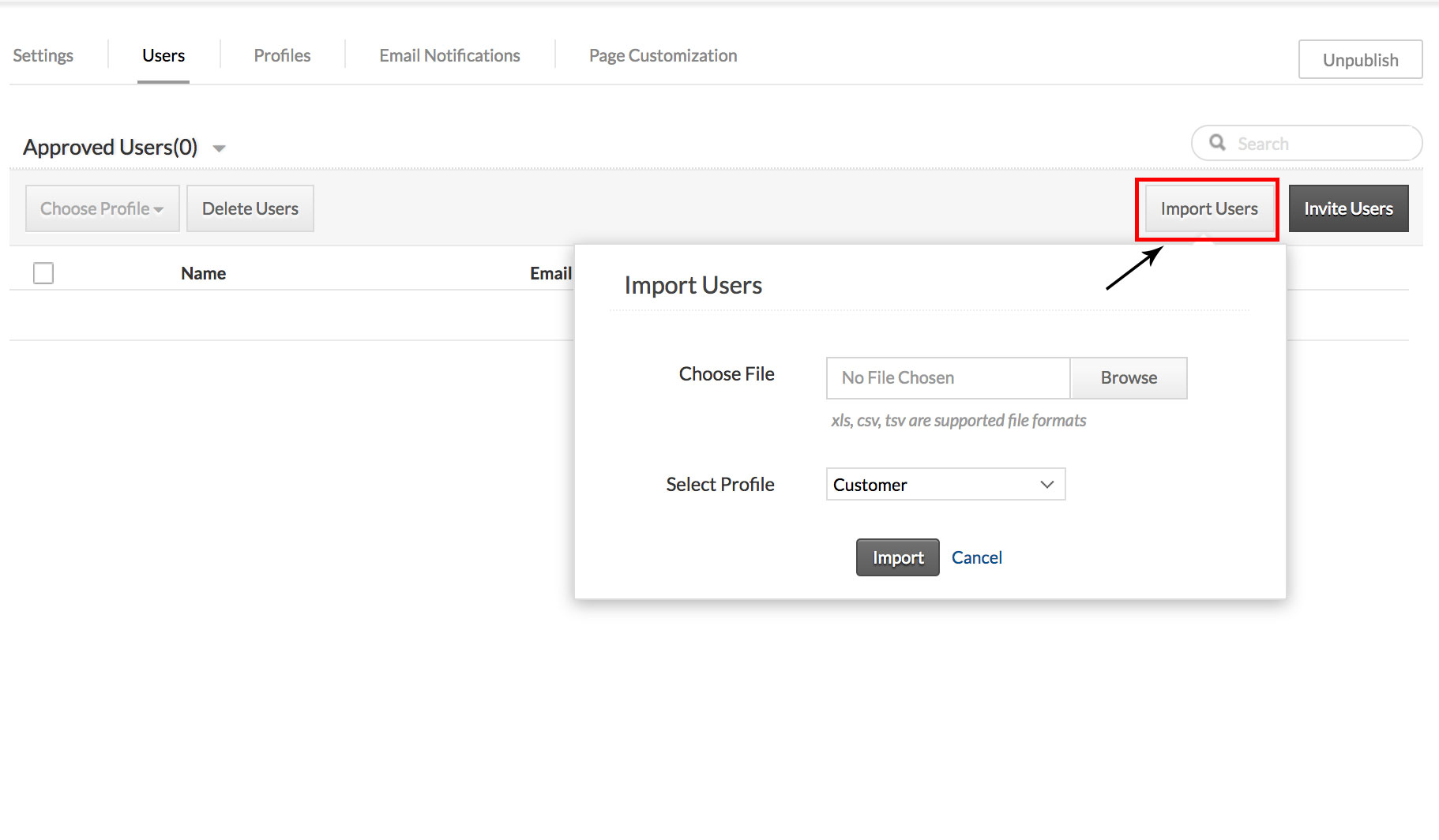In this image, there is a light purple outline surrounding a white background. At the top of the frame, there are several tabs including "Settings," "Users" (which is underlined), "Profiles," "Email Notifications," and "Page Customization." On the right side of this row, the word "Unpublished" is displayed.

Below these tabs, there is a section labeled "Approved Users," which currently indicates zero approved users. A downward arrow button is located next to this indicator, suggesting a dropdown menu. To the right of this, there is a search bar.

Further down, there is a light purple box containing various buttons. One button is labeled "Choose Profile," another is "Delete Users," and a third one, outlined in red, is labeled "Import Users." This "Import Users" button has been clicked, revealing a dropdown menu. The menu includes options like "Import Users," "Choose File" with an adjacent "Browse" button, "Select Profile" with a dropdown menu listing "Customer," and buttons for "Import" and "Cancel."

Below this dropdown menu, there is a line with small boxes labeled "Name" and "Email," followed by additional boxes underneath for user input.